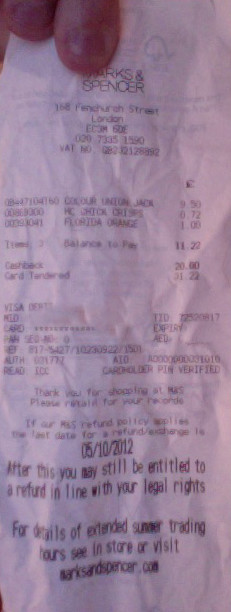This is a close-up image of a receipt from the store Marks and Spencer, held up in the top left corner by a person's fingers. The receipt is printed on very thin white paper, allowing some ink from the other side to be visible through the paper at the top and towards the middle. The receipt prominently displays "Marks and Spencer" at the top, although a finger is partially obscuring the "M" in Marks. Below the store name, the address is listed. The middle section of the receipt includes some credit card information. The total amount is $31.22, and towards the bottom, it mentions a date of 5-10-2012, followed by bold text about return policy information: "You may still be entitled to a refund in line with your legal rights." Additionally, it provides information about extended summer trading hours with a website link, www.marksandspencer.com.